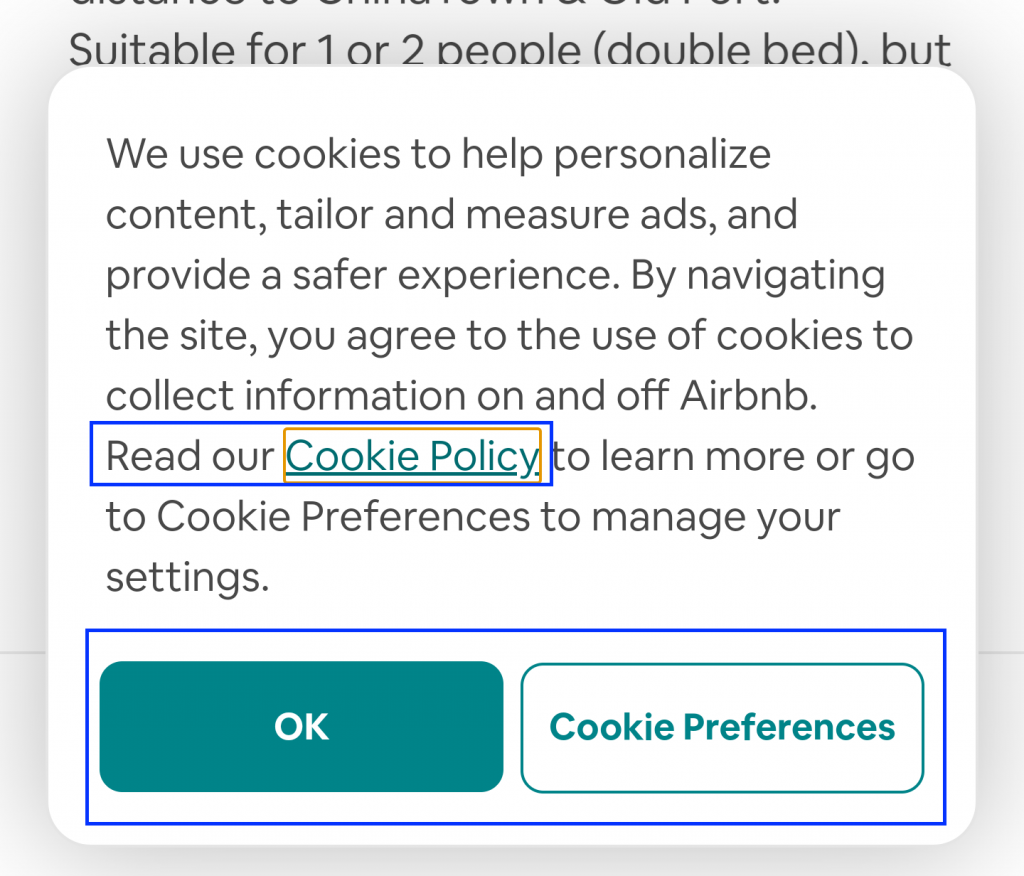The image prominently features a pop-up notification that covers most of the screen. The background of the pop-up is white and black. The text reads:

"We use cookies to help personalize content, tailor and measure ads, and provide a safer experience. By navigating the site, you agree to the use of cookies to collect information on and off Airbnb."

Highlighted within a blue box, the word "Read our" is displayed in black text, followed by "cookie policy" in green text with an underline, indicating a hyperlink. The phrase "cookie policy" is also enclosed in an additional green box.

Following the notification text, instructions in black text advise users to "learn more or go to cookie preferences to manage your settings."

At the bottom of the pop-up, there are two rectangular buttons: 
- The first one is teal with the word "OK" in white.
- The second one is white with the words "Cookie Preferences" in teal, each word starting with a capital letter.

Both buttons are outlined with a blue border.

In the background of the image, partially visible text reads: "Suitable for one to two people, double bed."